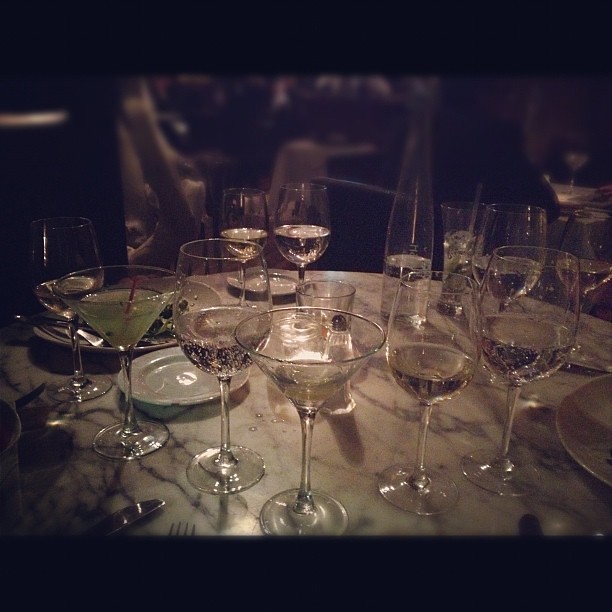The photograph captures a dimly lit dining table, likely situated in a restaurant or club, adorned with a variety of glassware. The table, covered with a white tablecloth, is crowded with a dozen glasses including martini, wine, and regular water glasses. Intriguingly, while most of the photograph is in black and white, one martini glass contains a noticeable green liquid, contrasting with the light-colored liquids in the other glasses, which could be water or sparkling water. A bottle of still water, partially filled, is placed towards the left middle of the scene. Eating utensils such as forks and knives, along with plates, are scattered around the table. Additionally, there's a visible salt shaker and minor spills of liquid on the tabletop. The background features blurred hints of more tables and chairs, suggesting the presence of other patrons. This detailed composition highlights the remnants of a possibly convivial gathering.